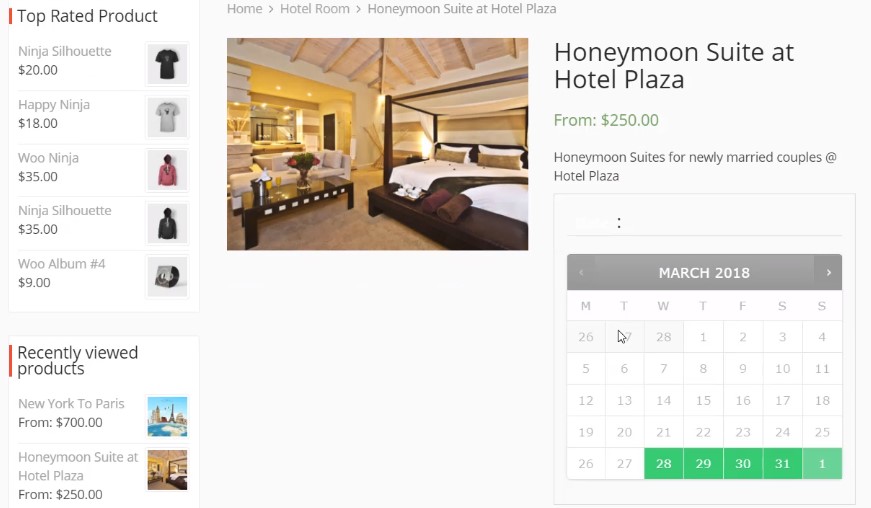The image displays a selection of top-rated products, prominently featuring:

1. "Ninja Silhouette" priced at $20
2. "Happy Ninja" available for $18
3. "Woo Ninja" offered at $35
4. Another product named "Ninja Silhouette" also sold for $35
5. "Woo Album Number 4" priced at $9

Additionally, it highlights recently viewed products which include:

- Flights from New York to Paris starting at $700
- Stays at Honeymoon Street at Hotel Plaza starting from $250

The image also has navigation links such as "Home," "Hotel Room," and "Honeymoon Street at Hotel Plaza" with the price starting from $250 for newly married couples. There is a small calendar marking the 28th to the 1st in green, whereas the rest of the dates are in white.